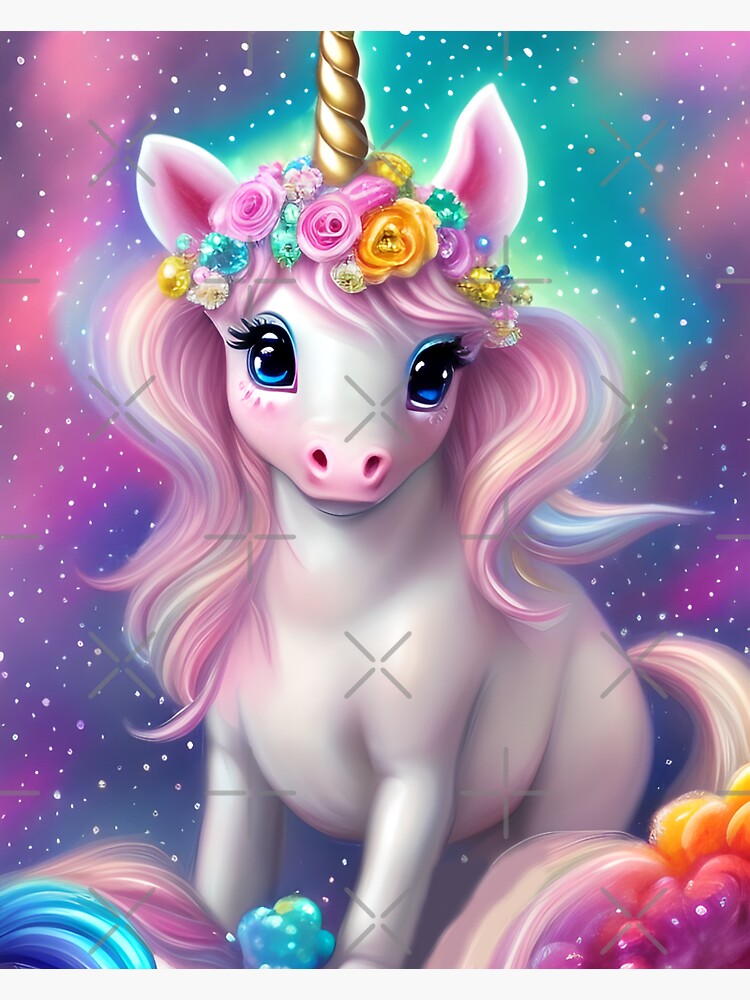This image is a highly detailed, colorful digital fantasy illustration of a tiny, light pinkish-white unicorn with big blue eyes and long black eyelashes. The unicorn's notable features include a golden horn adorned with a crown of flowers, which cascade into its multicolored mane composed of shades of pink, purple, blue, yellow, and green. The unicorn also has a similar vibrant tail, reflecting its rainbow-like hair. It stands against a galaxy-like backdrop that is dark interspersed with hues of pink, purple, green, and blue, dotted with white speckles to emulate a starry night. Further accentuating the magical setting are rainbow-colored edges featuring vibrant shades of purple, pink, green, and yellow, along with additional orange and lavender bubbly forms below the unicorn. Throughout the poster, tiny silver or gray X's are scattered, adding an intriguing layer to the artwork.